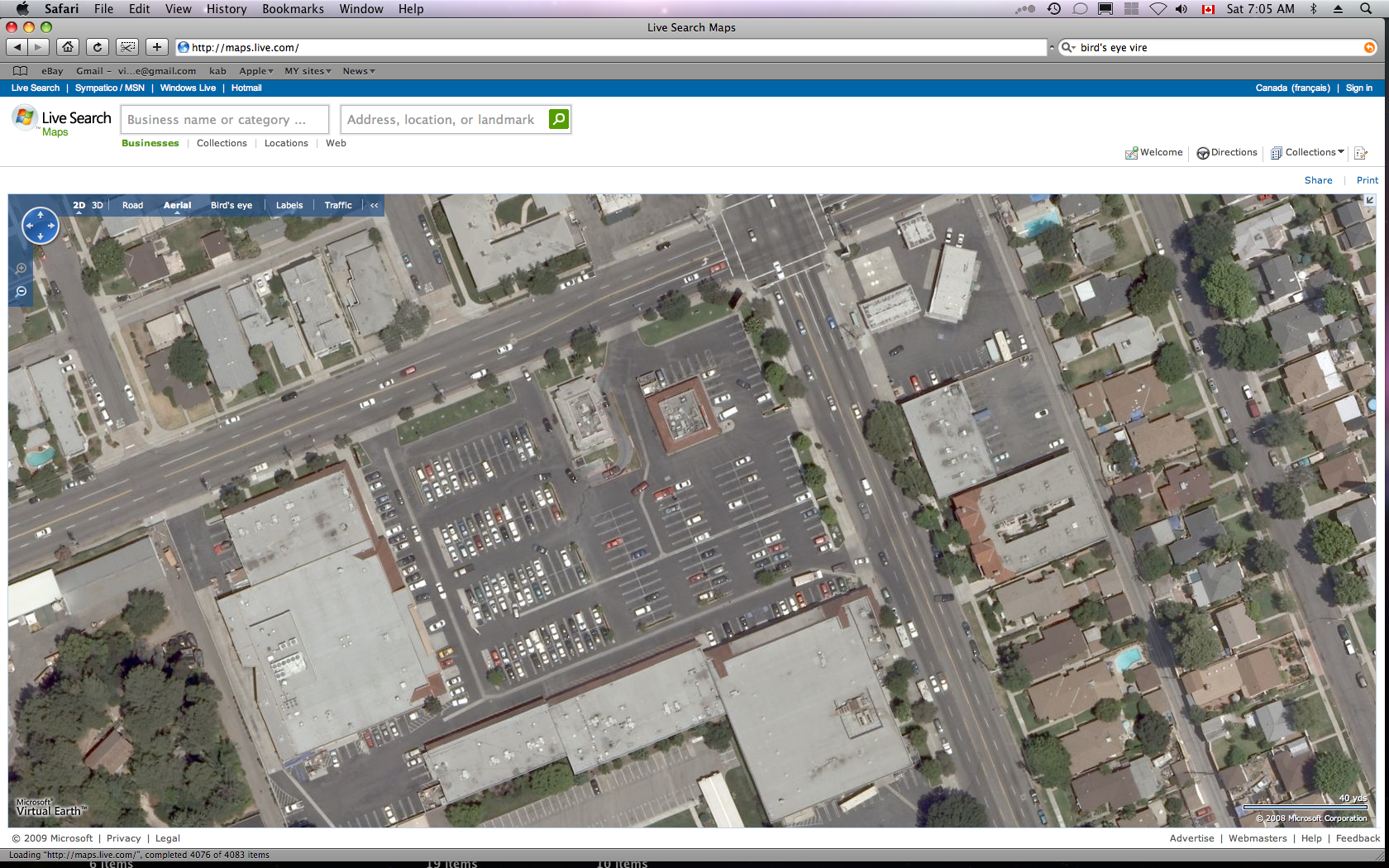The image depicts a screenshot of a Mac desktop with the Safari browser open. At the top, the iconic Mac Safari toolbar is visible, beginning with the Apple logo. Adjacent to it, Safari offers several menu options including File, Edit, View, History, Bookmarks, Window, and Help. On the right side of the toolbar, small icons indicate the computer's battery status, Wi-Fi connectivity, volume, and current time.

Beneath the toolbar, the silver Safari bookmark bar is displayed, featuring a white search and URL field currently set to http://maps.live.com. The webpage itself has a white border at the top, housing a search function that allows users to search by business name, category, address, location, or landmark. A "Live Search" button accompanied by a Windows icon is also prominent.

The main content of the webpage is an aerial map view reminiscent of Google Earth. The map reveals a suburban area centered around a large parking lot with black asphalt. The lot is bustling with parked cars and is bordered by a substantial building—likely a supermarket—distinguished by its tan, light grey roof and brown facade. Surrounding this central area, several rows of suburban houses are neatly aligned in three distinct rows.

On the left side of the map, adjacent to the parking lot and supermarket, a small forested area with dense tree coverage is visible. Additional trees are scattered throughout the neighborhood, lining some streets and properties, adding green patches to this suburban block. The general impression is an overhead view of a lively suburban community.